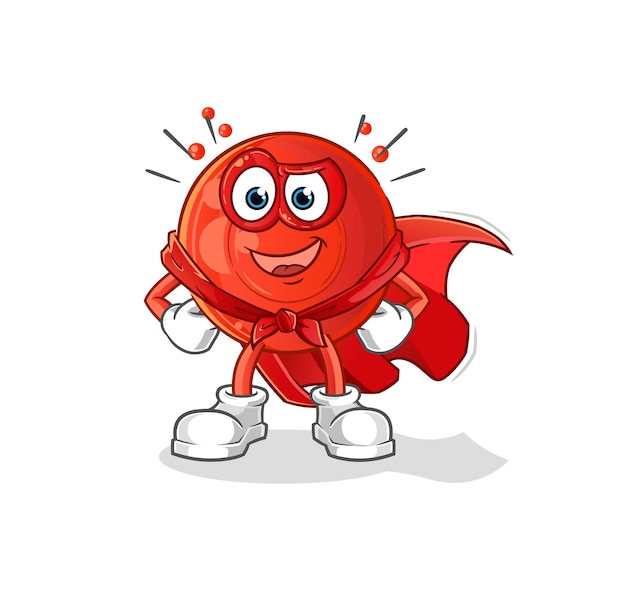The image showcases a vibrant, animated cartoon character set against a solid white background. The character is a bright red circle with a distinct superhero appearance. It features large white eyes with blue pupils framed by red eyelids, and a cheerful smile that reveals a red tongue. The character is adorned with red arms and legs, both ending in white gloves and white shoes respectively. Adding to its heroic theme, it wears a red cape tied around its neck, which flows behind it. Black stripes and yellow circles emanate from the top of its head, adding a dynamic and energetic feel. The character stands in a confident pose with hands on hips and legs spread apart, as if ready to take action.